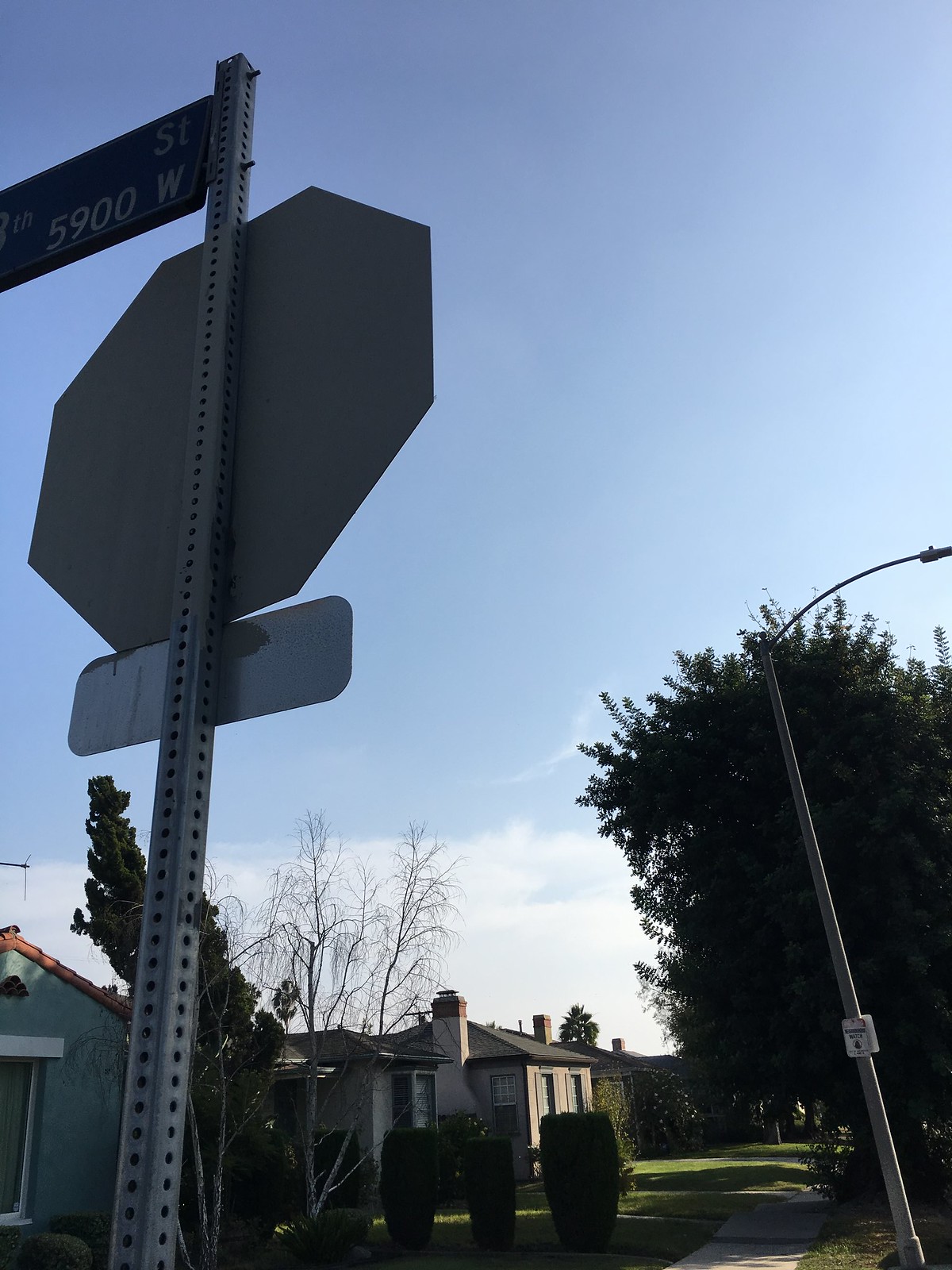In this photograph taken in a residential neighborhood on a bright afternoon, the foreground is slightly shadowed despite the clear blue sky dotted with clouds near the horizon. The first prominent element on the left is the back of a stop sign, beneath which another indistinguishable sign hangs. A partial street sign reading "5900 W Street" is visible, and to the right is a streetlamp standing in front of a large tree.

The scene unfolds along a residential sidewalk flanked by well-maintained houses. The nearest house on the left is beige with a visible chimney. Adjacent to it on the right is a brick house, also featuring a chimney. The house directly behind the street sign is blue with a distinct red tin roof and large, well-manicured cylindrical bushes—five in total—adding to its charm.

Further along the street, another house emerges, surrounded by leafless trees, hinting at the onset of spring or perhaps a clear, sunny winter day. Sunlight casts tree shadows onto perfectly green lawns, enhancing the scene of a well-kept and serene neighborhood.